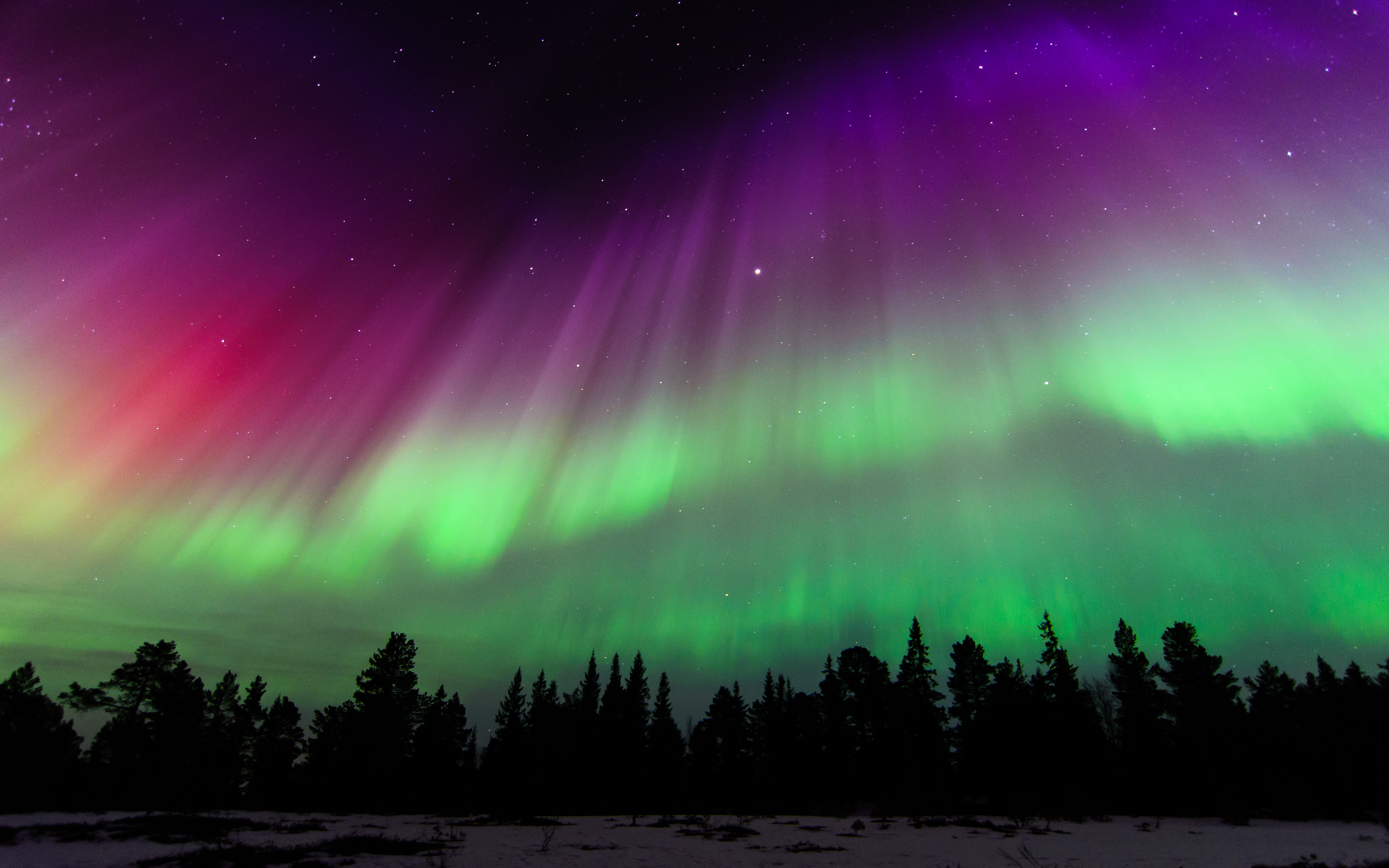A stunning photograph captures the ethereal beauty of the Aurora Borealis on a clear night. The foreground features a snowy landscape with a silhouette tree line dominated by pointed pine trees. Above this, a mesmerizing display of colors unfolds, beginning with a smoky, dark green band hugging the horizon. Ascending from this, vibrant streaks of lime green, pink, magenta, red, and purple radiate outwards from a dark blue or charcoal gray center at the top of the sky. The light source behind this center casts rays of shimmering colors that illuminate the heavens, with stars twinkling through the surreal light show. The entire scene stands out vividly against the black silhouettes of the trees, creating a stark yet beautiful contrast that highlights the extraordinary phenomenon of the Northern Lights.